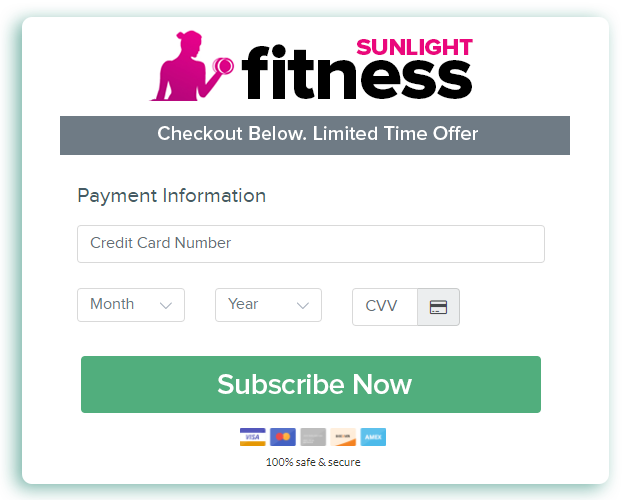### Descriptive Caption:
The screenshot showcases a webpage or mobile app interface designed for placing an order, presumably with Sunlight Fitness. The layout centers around a prominent white square outlined by a subtle light green glow, set against a white background. At the top, the logo for Sunlight Fitness is displayed prominently. "Sunlight" is written in bold, red, uppercase letters, while "Fitness" is in black, lowercase letters. Accompanying the text is a red silhouette of a person lifting a dumbbell, with a ponytail or bun depicted atop their head. Notably, "Sunlight" overlays the last three letters of "Fitness."

Just below the logo, a grey bar stretches across the screen. It contains the message in white text: "Check out below, limited time offer," with the acronym "CBLTO" capitalized. Further down, there is a section labeled "Payment Information" in capital letters, followed by a placeholder for the user to enter their credit card number. Adjacent to this input field are smaller boxes for the card's expiration month, year, and CVV code, with a visual cue of the card's back to assist users.

At the bottom of the form, a green bar with the text "Subscribe Now" invites users to complete their subscription. Below this call-to-action are various credit card logos, including Visa, MasterCard, a grey card (possibly a Platinum Amex), an unidentified card, and a Blue Amex. The footer reassures users with the phrase "100% safe and secure," emphasizing the site's commitment to security.